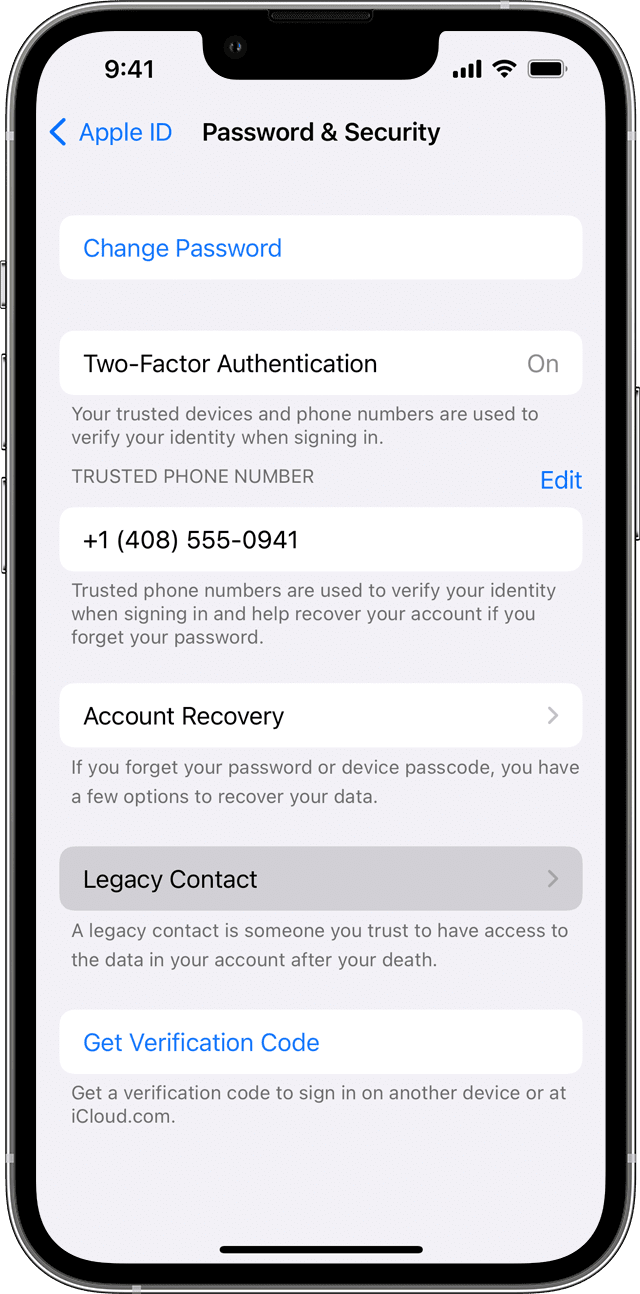A close-up, high-resolution image features an iPhone with a black bezel and visible silver edges against a white background. At the top center, the iPhone's notch is clearly visible, housing the front camera. The screen displays a settings page for Apple ID, focusing on Password and Security settings. The time reads 9:41 AM in black, positioned at the upper left corner, while the upper right corner shows icons for full cellular signal, full Wi-Fi signal, and a fully charged battery.

Below these elements, the interface displays a back arrow in blue pointing to the left, labeled "Apple ID." The main content includes a section titled "Password and Security," offering a blue button to change the password. It also describes Two-Factor Authentication as "On," noting that trusted devices and phone numbers are used for identity verification during sign-in. Below this, a trusted phone number, +1 (408) 555-0941, is shown with an option to edit in blue text.

Further details include descriptions related to Account Recovery, instructing users on options available if they forget their password or device passcode. There's a section on "Legacy Contact," explaining that this feature allows a trusted person to access the user's account data after their death. A blue button labeled "Get Verification Code" offers additional security options, with a brief explanation beneath it about obtaining a code for signing into the Apple ID or iCloud.